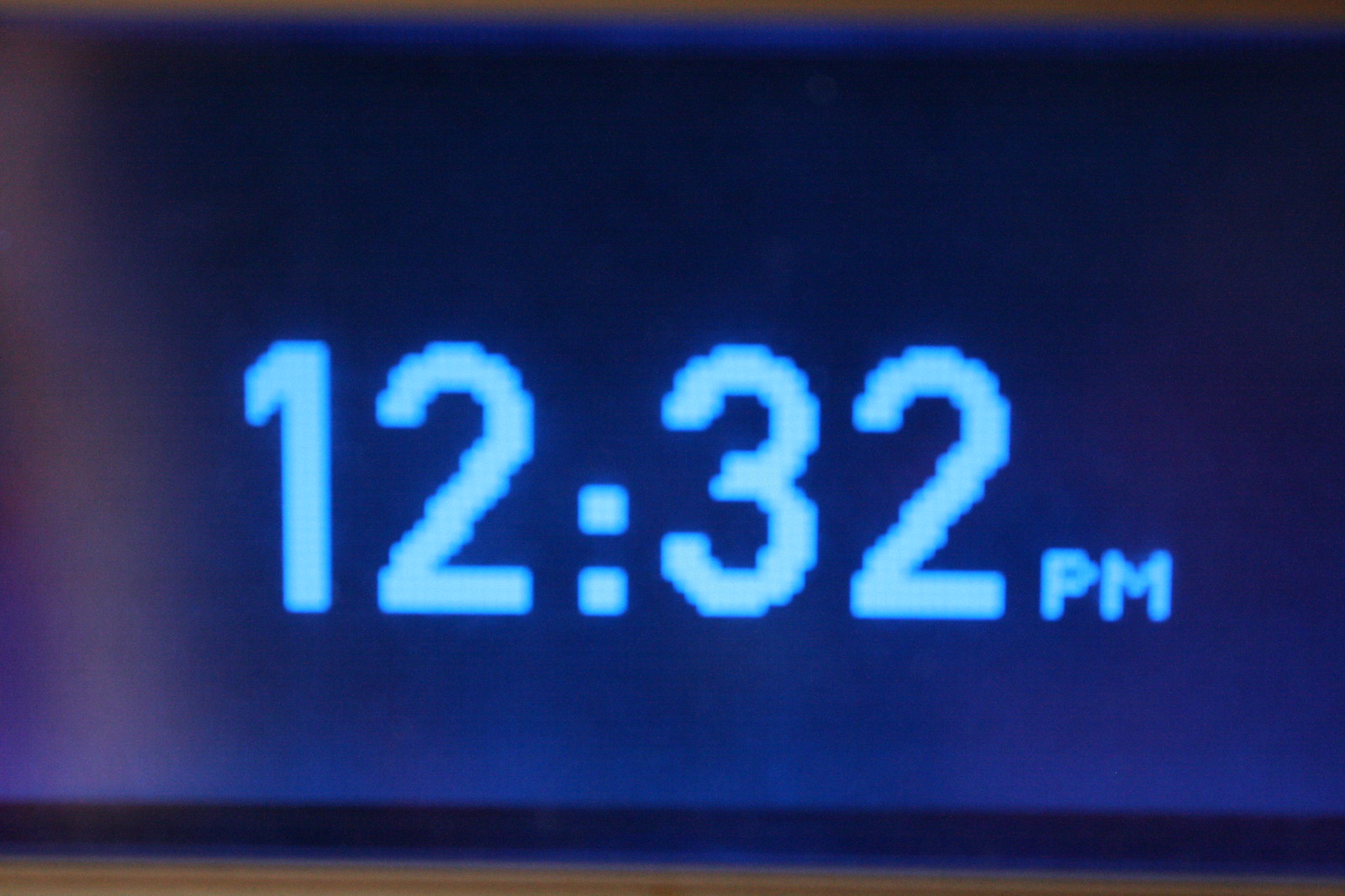This is a close-up image of a digital clock displayed on a blue background with wood framing the top and bottom. The clock reads 12:32 p.m., with the digits appearing in a light blue color and surrounded by a slightly darker blue outline. Each digit has specific characteristics: the '1' is straightforward and straight-edged, the '2' is slightly jagged with a puffier appearance at the top, the middle dots are small squares with a lighter image inside, the '3' shares the same jagged edges as the '2', and the final '2' mirrors the first. The letters "p.m." are in straightforward, capital letters. The darker blue framing around the numbers creates a distinct contrast, central to the image, giving a clear depiction of the time.